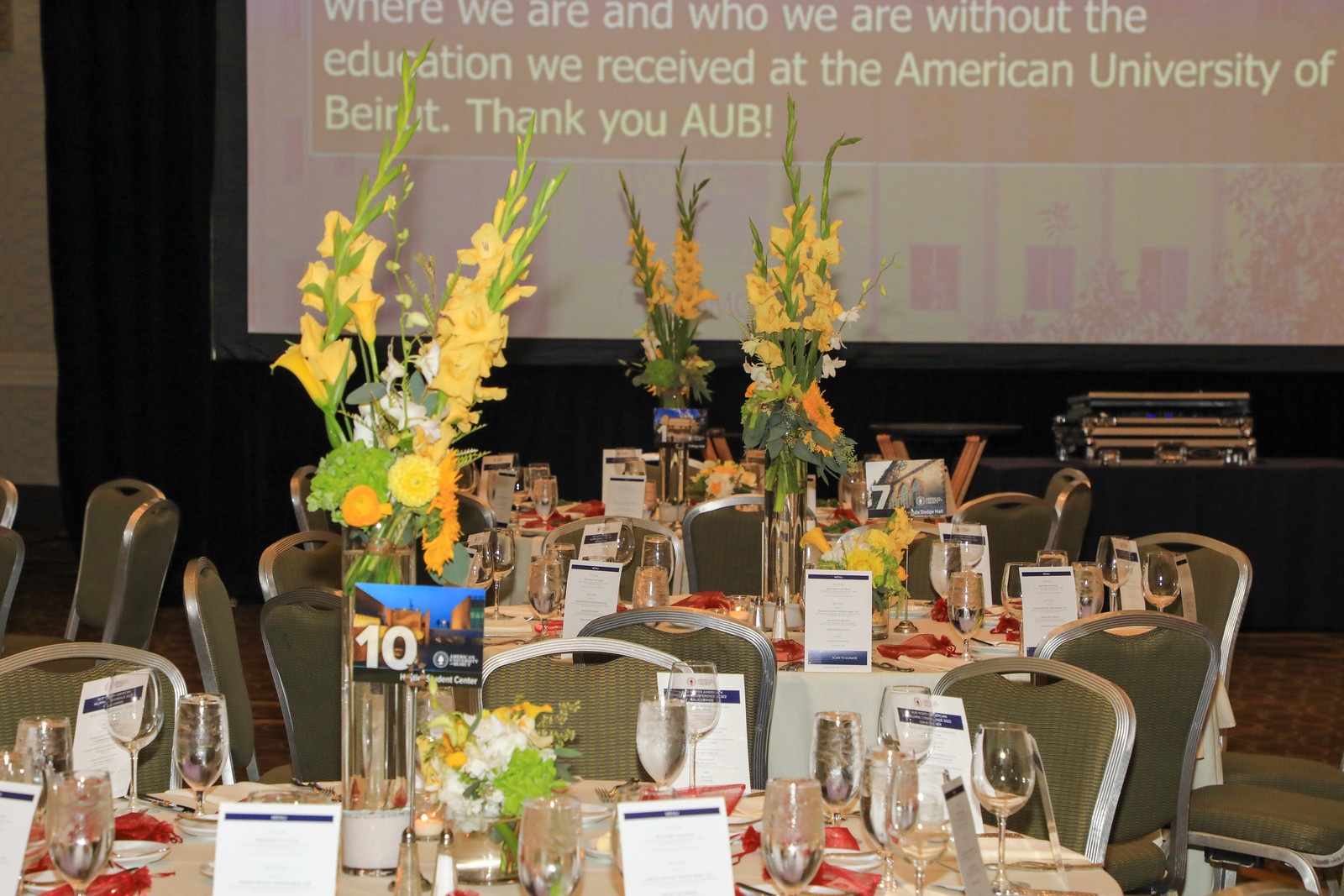The image depicts a well-appointed banquet hall featuring several round tables adorned with elegant place settings, complete with stemmed glassware, red napkins, and menu cards. Each table showcases tall glass vases filled with vibrant yellow, orange, and white flowers as centerpieces. The chairs surrounding the tables are green with silver frames, complementing the white tablecloths. In the backdrop, a large projector screen displays a message: "Where we are and who we are is without the education we received at the American University of Beirut. Thank you AUB!" The screen also includes some smaller, indistinct photos beneath the text. In front of the screen, a stage is set with what appears to be a silver case and additional seating arrangements. The meticulous arrangement and decor indicate a formal and celebratory event.